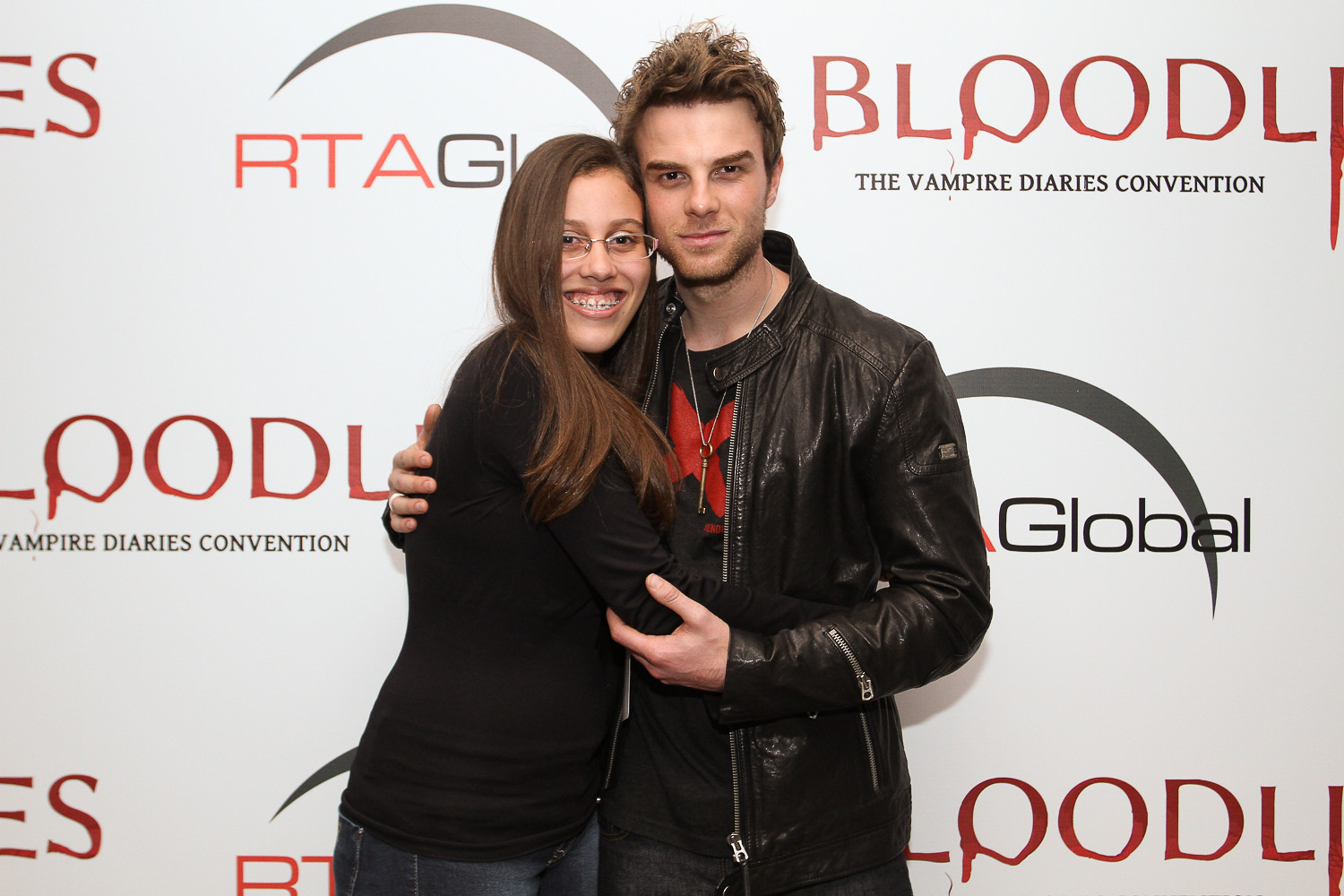At a vibrant red carpet event, a large backdrop captures attention with its white background adorned with various logos and partially visible text including "Blood, Blood, Blood Leaves" and a tagline that reads "The Vampire Diaries Convention." The back of the banner also showcases the logos of "RTA Global." In front of this backdrop stand two individuals engaged in a heartfelt embrace. On the left, a woman appears with her glasses, braces, black sweater, and blue jeans. She is being embraced by a man to her right, who sports a black leather jacket, a black tee with a red cross design, black jeans, and a spiked hairstyle. His arm lovingly wraps around the woman's back while his other hand gently touches her right elbow as she hugs him. The scene is framed with a sense of warmth and camaraderie amidst the glitz of the event.